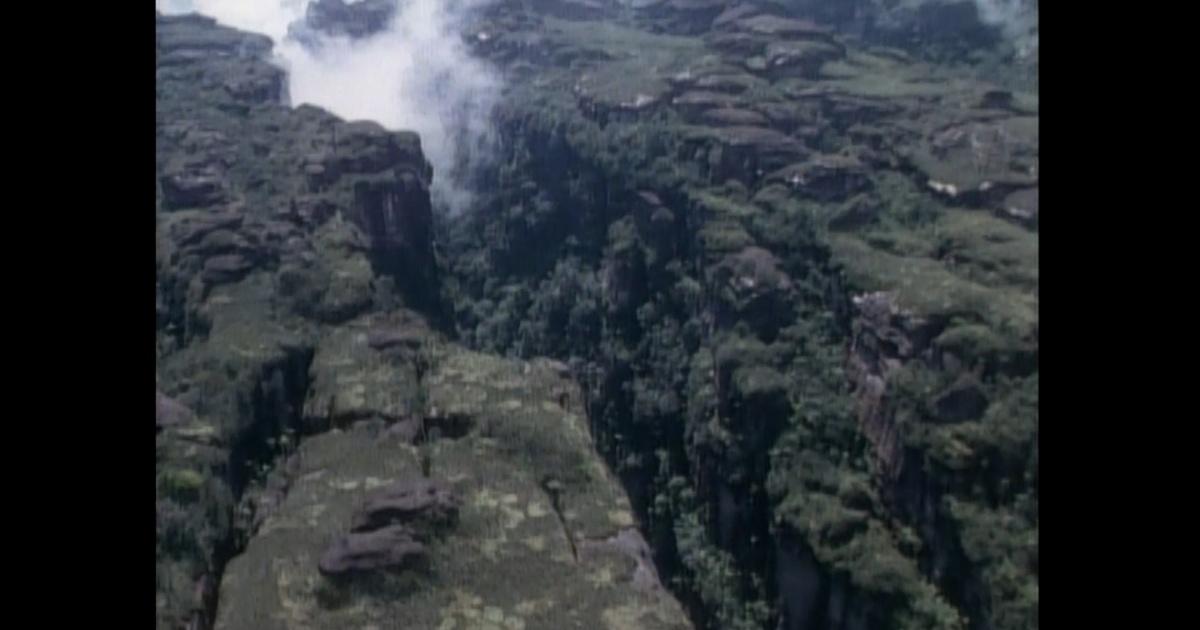This photograph provides a sweeping aerial view of a steep, v-shaped canyon that spans diagonally across the image from right to left. On either side of the canyon, the dark rocky walls exhibit patches of vibrant green moss, while scattered bushes and trees cling to the rugged landscape. Toward the top of the image, a thick mist or smoke rises, partially obscuring the canyon walls and softening the vivid colors of the rock and vegetation. The bottom of the canyon remains hidden, though glimpses of white spray suggest powerful ocean waves crashing into the cliff walls. The entire scene is presented through the frame of two thick, black vertical bars on either side, making the vista seem like it's viewed from a narrow, focused perspective. The image, though slightly blurred, captures the dynamic and dramatic interaction between land and sea, rock and mist.